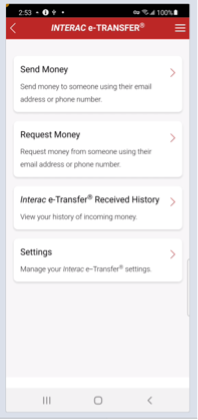This screenshot captures a mobile banking application interface. The top section of the screen is characterized by a black status bar that displays the time as 2:53, alongside icons for Wi-Fi, carrier signal strength, and a fully charged battery at 100%. Below the status bar, a red banner features a back arrow on the left, the title "Interact e-Transfer" centered, and three white lines (likely a menu icon) on the right.

Beneath the red banner, the main body of the interface is divided into distinct sections. At the top, a box labeled "Send Money" is accompanied by a red arrow pointing to the right. The description under this box instructs users to send money to someone using their email address or phone number. 

Following that, another box labeled "Request Money," also with a red arrow to the right, explains how to request money from someone through their email address or phone number.

Further down, there is a section titled "Interact e-Transfer Received History," which allows users to view their transaction history, including received amounts and other relevant details. The final section is "Settings," which provides access to manage Interact e-Transfer settings.

The interface is organized and user-friendly, designed to facilitate easy navigation for sending, requesting, and managing money transfers via email or phone number.